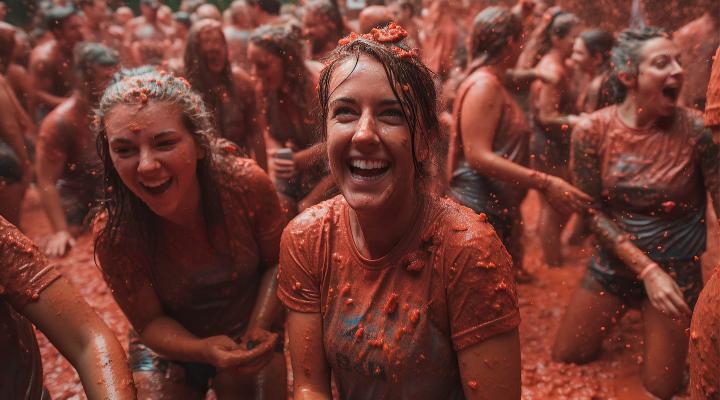This vibrant image captures the exuberant chaos of the famous tomato festival in Spain, where revelers immerse themselves in a jubilant tomato fight. Mostly women, though some men are present, stand in a knee-deep pool of reddish-orange tomato mush that extends far beyond the visible frame. Dressed in shorts and t-shirts now completely covered in clumpy tomato residue, participants' laughter fills the scene. The central focus is a brown-haired woman with wet bangs partially draped over her face. Her eyes are squinted with a wide smile, exposing her top teeth as she shares the joy of the moment. To her right, another woman bends forward in laughter, likewise drenched in tomato pulp. Most faces sport remnants of the pulpy sauce, and the blurred background reveals clusters of merrymakers, surprised and delighted in equal measure by the messy festivities.